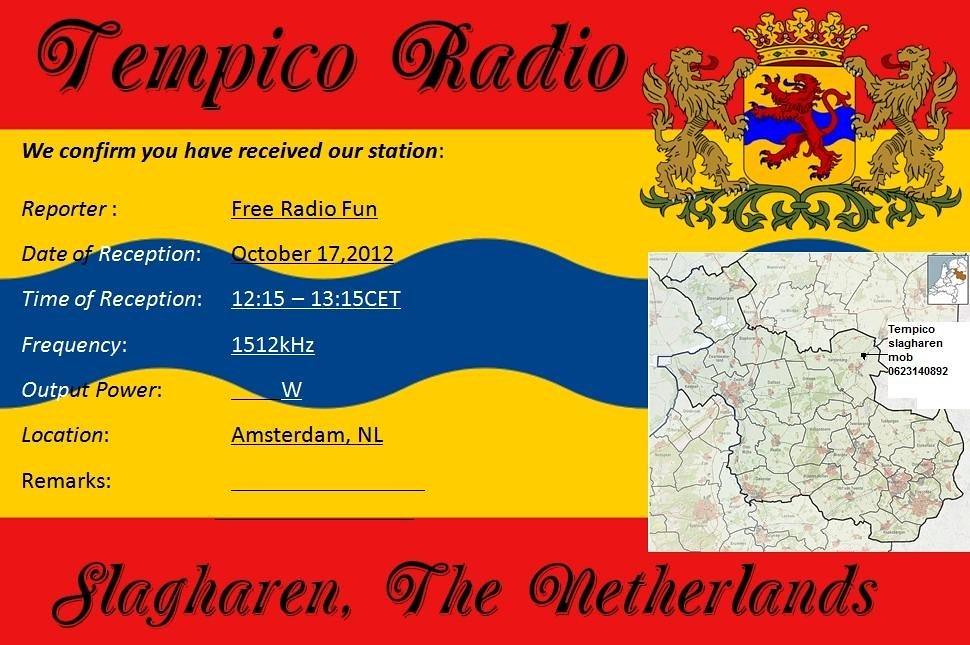This colorful poster celebrates the recognition of a radio transmission received. Dominated by dark red bands at the top and bottom, the central two-thirds of the poster features a vibrant yellow background. In the top left corner, black letters spell out "Tempico Radio," adjacent to a detailed crest on the right. The crest showcases two lion-dragon hybrid creatures in light greenish-yellow, standing on their hind legs with tongues protruding. They hold a shield displaying a similar figure with a dark blue-purple tongue, and a yellow crown adorned with jewels sits atop the shield.

Below "Tempico Radio," the yellow background features blue letters stating, "We confirm you have received our station." Additional details include "reporter: Free Radio Fun, date of reception: October 17, 2012, time of reception: 12.15 to 13.15 CET, frequency: 1512 kilohertz," and "location: Amsterdam, NL."

On the right side, there is a white insert with a black-outlined map of the Netherlands pinpointing the location. At the very bottom, the red banner includes black lettering that reads, "Slagharen, the Netherlands."